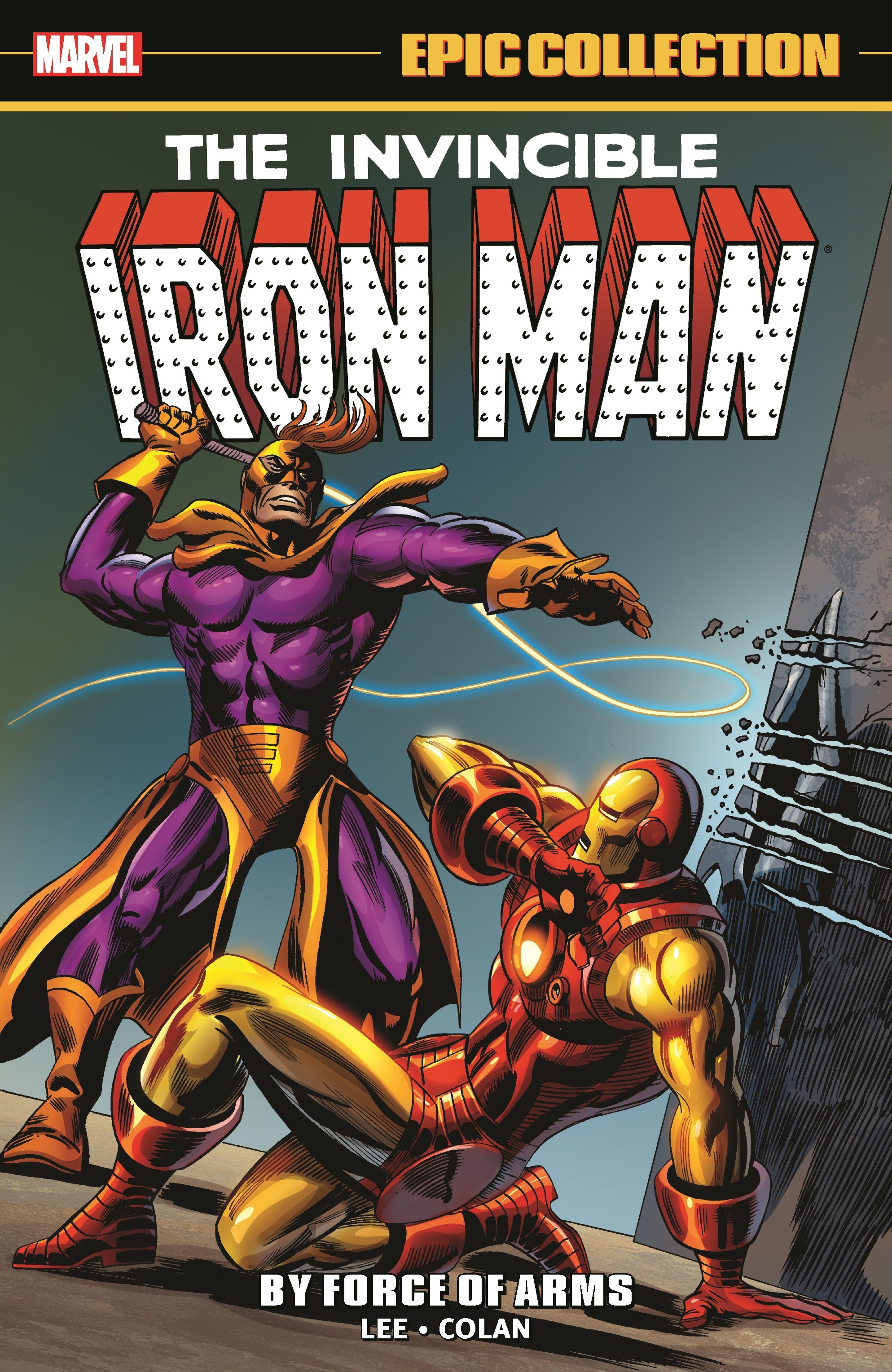This vivid and detailed comic book cover features a black border at the top with a gold line beneath it, and in bold gold letters, it reads "Epic Collection." In the upper left corner, over a red rectangular background, "Marvel" is written in white. Just below the gold border, the title "The Invincible Iron Man" is displayed, with "Iron Man" rendered in bold, three-dimensional block letters—white-faced with red sides.

Central to the cover's illustration is a dramatic confrontation. Iron Man, clad in gold and red armor with a distinctive helmet, kneels in a protective, almost submissive posture, visibly distressed. The foreboding villain standing over him is dressed entirely in purple with striking gold accents, including a scarf, gloves, boots, and shorts with a flowing ribbon. The villain, muscular and menacing, wields a whip made of light, which arcs dangerously behind him.

Other background colors like black, white, brown, and blue enhance the vivid scene. Beneath this intense standoff, the text "By Force of Arms, Lee Colan" is prominently shown, signaling the creative minds behind this comic spectacular.